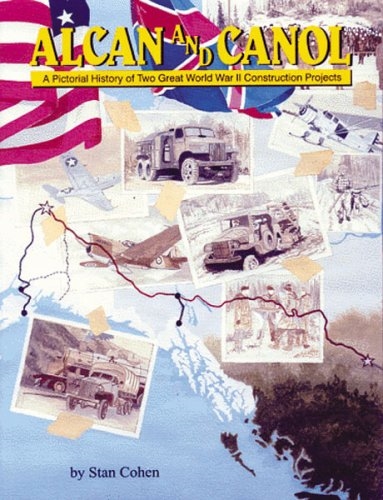The cover, resembling that of a hardcover book, possibly a pictorial history, prominently features the yellow headline "ALCAN and CANOL: A Pictorial History of Two Great World War II Construction Projects" set against a rich background. The layout includes a vibrant collage of historic World War II images, with army vehicles like trucks, Jeeps buried in mud, and aircraft equipped with skis. Artist's sketches depict soldiers in cold weather gear engaged in monumental tasks, emphasizing the rugged conditions. A map detailing routes from Alaska to Canada, framed by the snowy terrain, underlines the construction theme. Flags of the USA and Britain adorn the top left, along with borders and paths suggestive of military movements. At the bottom right, the book is credited to Stan Cohen.